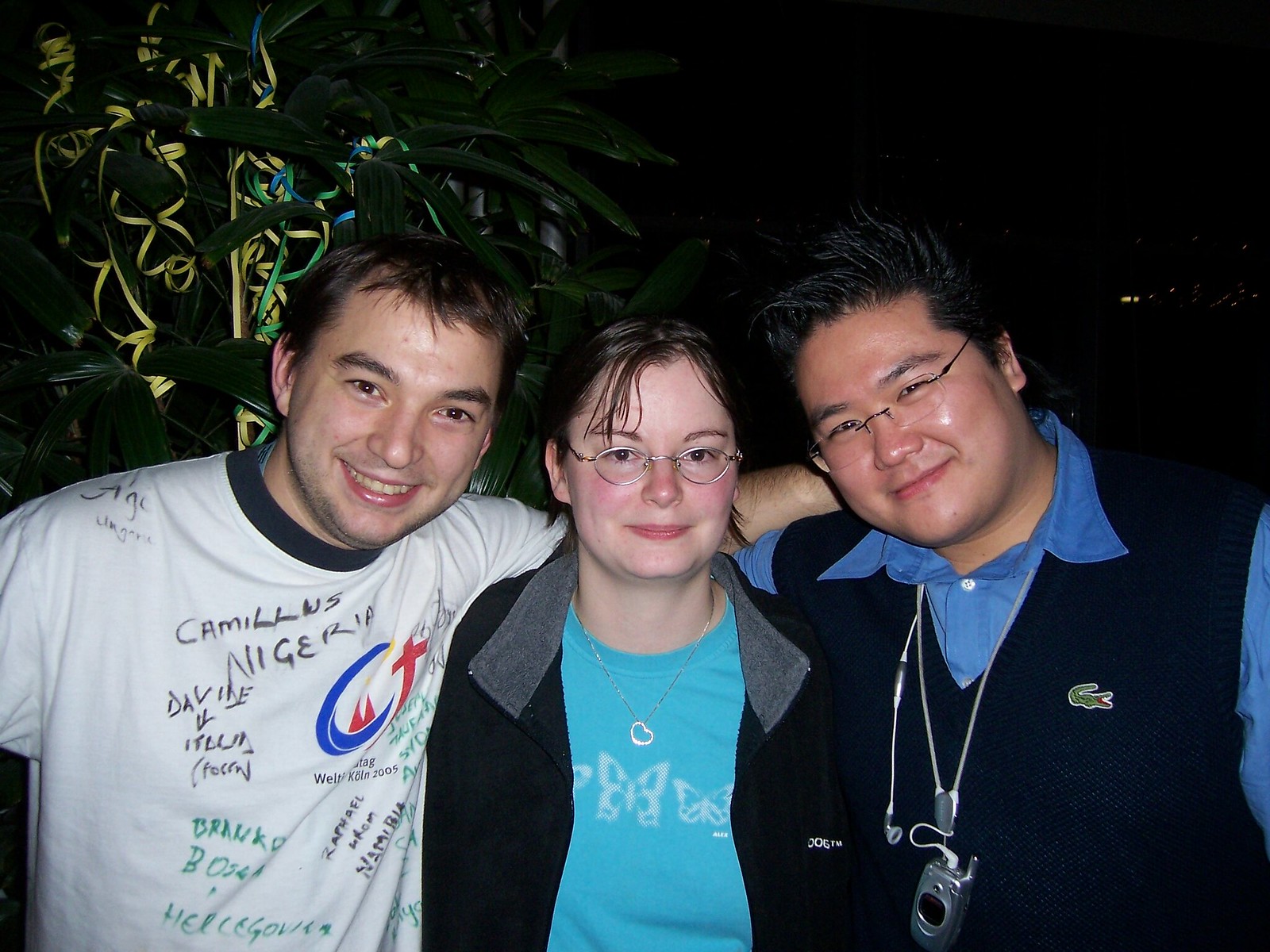In the image, three friends, who appear to be of Asian descent, are joyfully posing together against a black backdrop. Twirly ribbons hang down on the left side, adding a festive touch to the scene. 

On the right, a gentleman with dark hair and glasses is wearing a Lacoste black sweater vest over a blue shirt. He is smiling warmly. 

In the center, a young lady is donning an open black jacket that reveals a blue tee and a heart necklace. She, too, wears glasses and has short dark hair.

To the left, another gentleman, sporting a white tee with a blue logo featuring red sailboats, is grinning broadly. The camaraderie between them is evident, as they have their arms wrapped around each other’s backs, clearly enjoying this moment together.